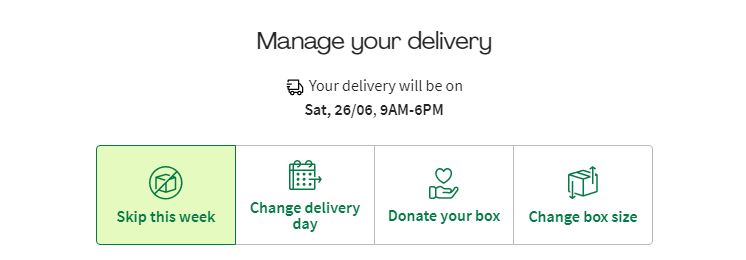The image showcases a delivery management interface. At the top, bold letters spell out "Manage Your Delivery." Below this heading, there is a simple black outline of a truck facing to the right. Directly beneath the truck icon, gray text reads, "Your delivery will be on: SAT, 26/06, 9 a.m. to 6 p.m."

Under this information, there are four options enclosed in outlined boxes:

1. The first box, bordered in a thin dark green line with a light green background, features an icon of a three-dimensional box with a slash through it. Centered below the icon, green text says, "Skip This Week."
   
2. The second box, with a thin gray outline and a white background, contains a green outline graphic of a calendar with an arrow pointing to the right. Below this icon, the green text reads, "Change Delivery Day."

3. The third box, also outlined in gray with a white background, displays a green-outline graphic of a hand holding a heart. The green text under this icon says, "Donate Your Box."

4. The fourth box, similarly outlined in gray with a white background, shows a three-dimensional box with an arrow pointing downwards and another arrow pointing upwards. Below this, in green text, it reads, "Change Your Box Size."

This image efficiently guides users through several options for managing their upcoming delivery.